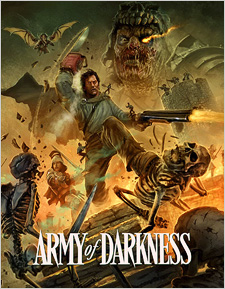The vividly detailed poster for "Army of Darkness" showcases its title at the bottom, with "ARMY" and "DARKNESS" in bold, capitalized white letters, and "of" in smaller lowercase. At the center of the dynamic scene, a man leaps through the air, gripping a sawed-off shotgun in his left hand, which fires with a visible spark. His right hand brandishes a chainsaw blade, slicing through a living skeleton on the left. Simultaneously, he kicks another skeleton with his left leg. Beside him, another man clad in ammunition fights with a sword. In the top left corner, a large, human-like creature with a glowing left eye looms menacingly near a tower. The scene is highly detailed, brightly lit, and filled with action, including three individuals shooting arrows at monstrous creatures. The overall image is colorful and clear, capturing an intense moment of combat.